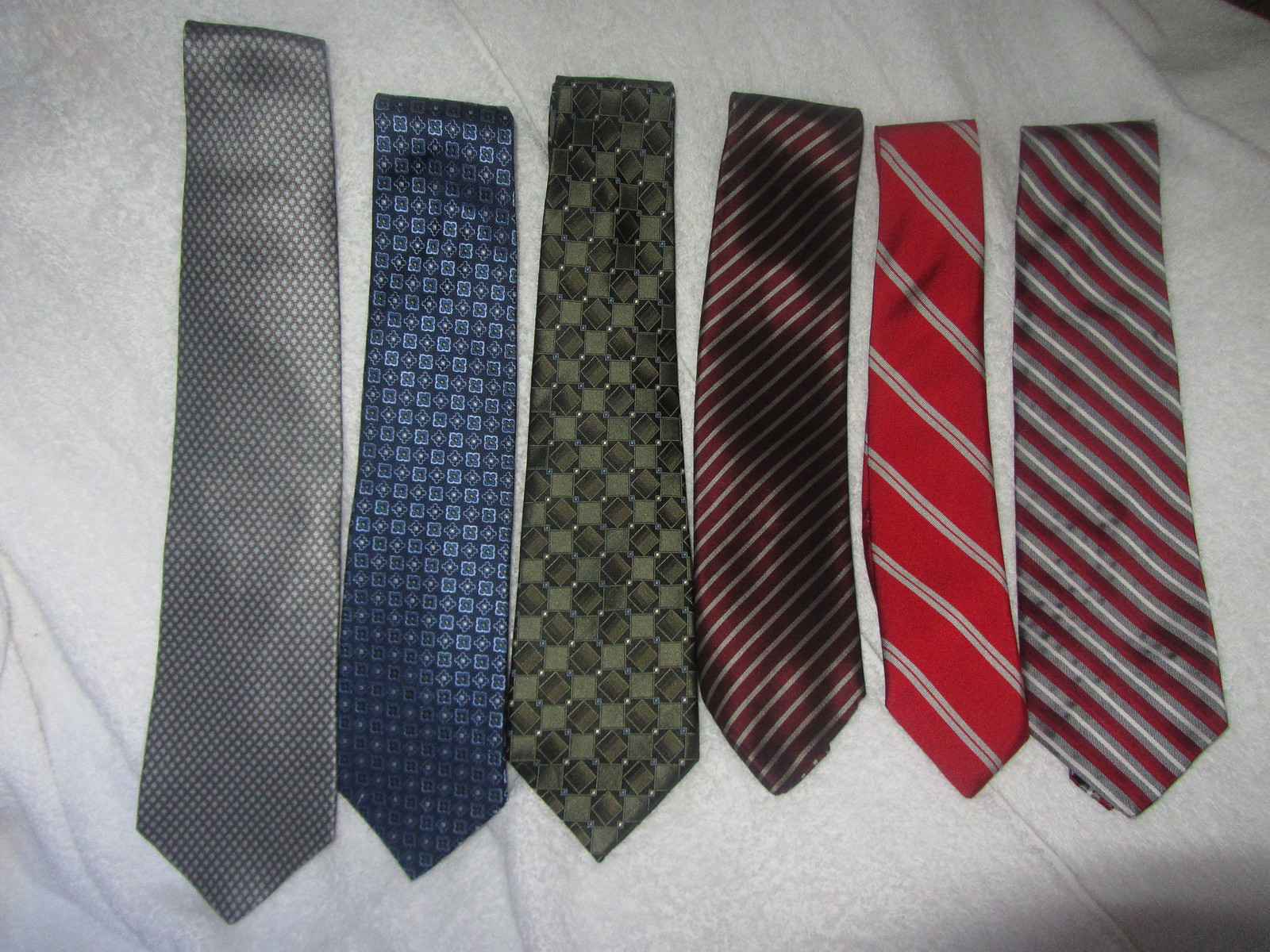This image features six silk neckties, meticulously folded to display their bottom color schemes, and arranged vertically from left to right on a white cotton backdrop. These ties exhibit a range of widths and lengths, each presenting a distinct pattern. 

From left to right:
1. A gray tie adorned with tiny, possibly star-shaped or diamond-shaped designs in black.
2. A navy blue tie featuring an alternating pattern of small blue squares and diamonds.
3. An olive green tie with a grid-like pattern of dark green and white squares and diamonds.
4. A dark burgundy tie with thin silver diagonal stripes running from the top right to the bottom left.
5. A bright red tie with wider-spaced, silver diagonal stripes going from the top left to the bottom right.
6. Another red tie, slightly darker, with silver and gray diagonal stripes closely spaced, creating a subtle contrast.

These ties, made from slightly shiny silk fabric, rest neatly on a white cloth, possibly a bed sheet, enhancing their vibrant designs and colors.